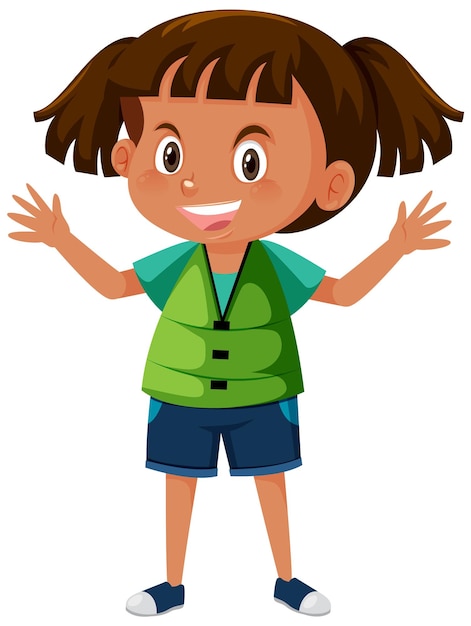This is a detailed digital drawing of an animated young girl who resembles Dora the Explorer, featuring a charmingly expressive demeanor. She has brown hair styled in pigtails with playful bangs, complemented by her warm tan skin and dark brown, almost black eyes. Her mouth is open, revealing her upper row of teeth as if she's in mid-sentence, adding to her lively expression. Her eyebrows are lifted, and she is holding her arms out to her sides with fingers splayed like jazz hands. Her outfit includes a teal-colored t-shirt beneath a green vest that resembles a life jacket, paired with blue denim shorts that have small rolled-up cuffs. Her legs are notably slender, contrasting with her relatively larger torso, and she wears blue shoes with white tips. The entire image is set against a simple, stark white background, accentuating the character's vibrant details.